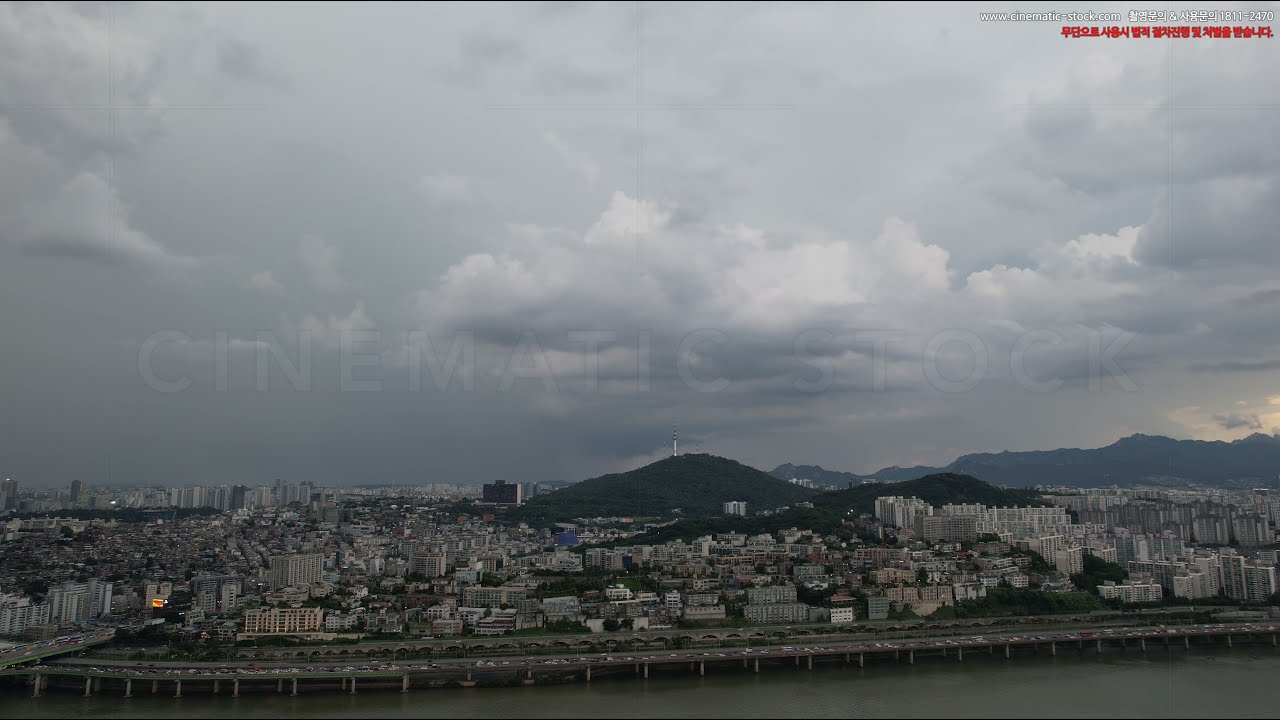The image is a full-color stock photo taken outdoors on a very overcast, dreary day, featuring a large city situated next to a body of water. The foreground of the image shows the water with a raised roadway on columns crossing over it, congested with cars. Behind the roadway, the cityscape unfolds with a mix of small, closely-packed apartment buildings and larger skyscrapers. The smaller buildings are centrally located, while taller, uniform-colored structures dominate the right side, and larger buildings are on the back left. A distinctive hill with green bush and a tall, cylindrical building resembling a lighthouse stands out in the center of the photo. Beyond it, a range of mountains can be seen. The background is filled with thick gray overcast clouds, adding to the gloomy ambiance of the scene. A watermark reading "Cinematic Stock" is present across the center of the image. There are no clear indicators of the city’s identity or the time of year.